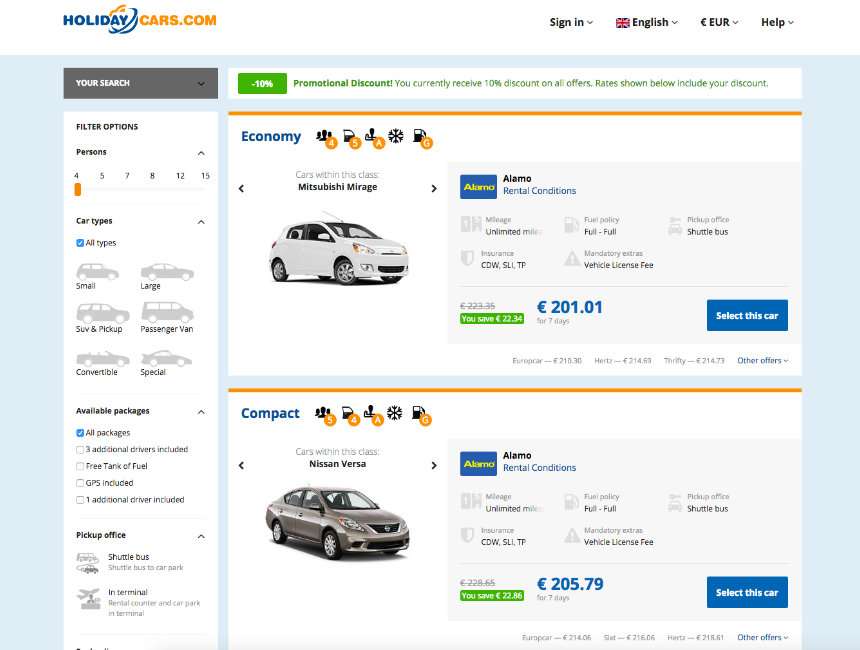The image depicts a section of a car rental search results page from HolidayCars.com. At the very top, "HOLIDAYCARS.COM" is prominently displayed, with "CARS.COM" in uppercase orange text. To the right, user options include "Sign In," "English," "EUR" for European currency, and "Help."

Below these options is a dark gray search bar with placeholder text that reads "Your Search." Adjacent to the search bar, there is a green rectangle highlighting a "10%" promotional discount alongside text that states: "You currently receive 10% on all offers. Rates shown below include your discount."

The first listing features a small white car classified under the "Economy" category from Alamo Rental Company. The price is marked at €201.01, and there is an option to "Select This Car" in a blue rectangular button.

The second listing shows a slightly larger four-door vehicle in a gray or silver color, labeled as "Compact." This vehicle is also from Alamo, indicated by the "Alamo" logo within a blue square, accompanied by the text "Alamo Rental Conditions." The price for this vehicle is €205.79, and a blue rectangular button offers the option to "Select This Car."

Both listings and their details are outlined in a light blue square, making the information visually distinct.